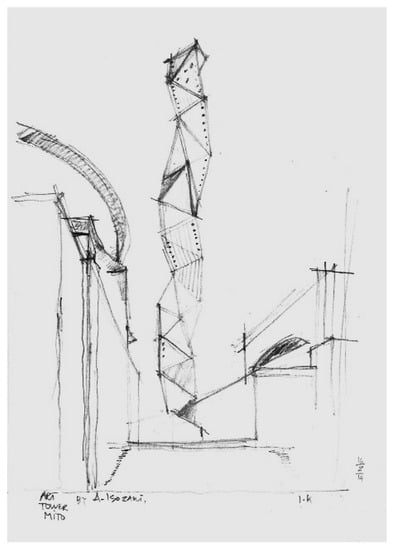This artwork appears to be a detailed black and white sketch titled "Art Tower MITD" by Alonza Nia or possibly A. Isozani, although the exact name remains somewhat unclear. The focal point of the piece is a tall, snake-like tower constructed from triangular forms that rise sinuously in the center of the drawing. Flanking the central tower are additional structures: on the left, a building or track-like feature, and on the right, what seems to be a staircase or possibly another building. The complexity of the drawing makes it somewhat challenging to decipher every element. The background is a clean white, emphasizing the stark black lines and shapes that comprise the mysterious and intriguing composition.